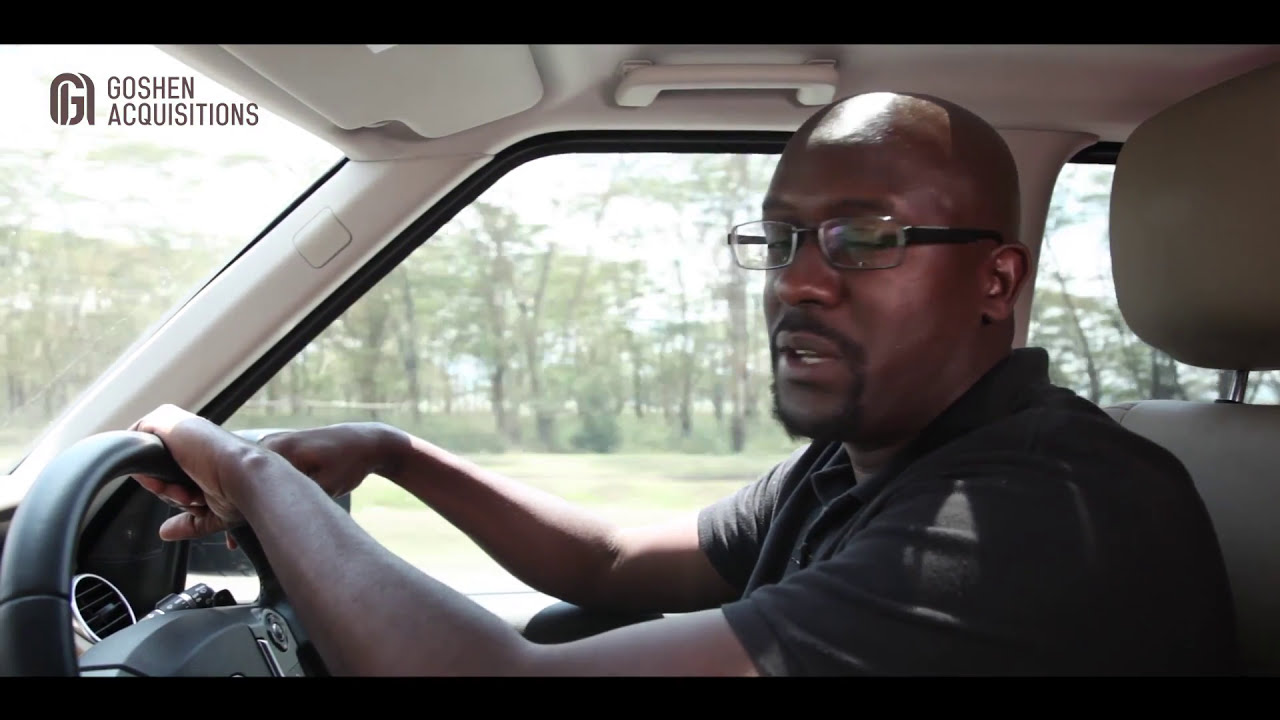The image depicts a black male driving a vehicle, with sunlight streaming through an open skylight, illuminating his receding hairline and short buzz cut. He is wearing wireframe glasses with black side supports, and he sports a mustache and a slight goatee. Dressed in a black polo shirt with short sleeves and a white logo on the sleeve, he has his hands on the steering wheel, positioned at the top and an arm resting to the side.

The interior of the car features a beige upholstery, with leather-like cushion seats and a black steering wheel. There's a grab bar above the door and visible vents on the left. On the top left corner of the image is the text "Goshen Acquisitions" alongside a logo where a 'G' intertwines with an 'A'. Through the passenger side window, and partially through the front, a rural landscape is visible, including a line of trees, grassy fields, and a sunny but slightly cloudy sky in the background. The man appears to be speaking into the camera, possibly for an infomercial or advertisement.